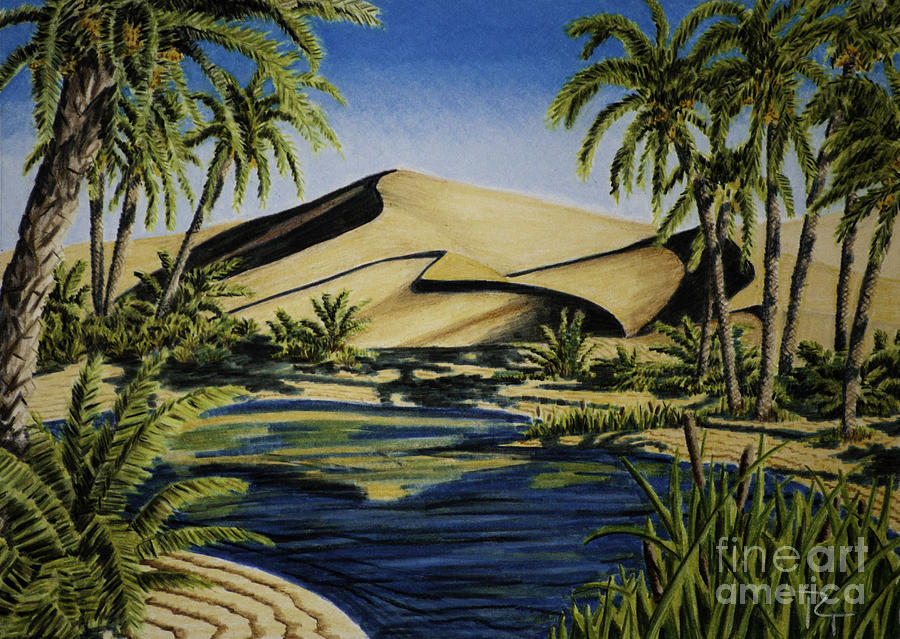This is a detailed painting of a vibrant desert oasis, featuring a striking blue body of water in the center. Surrounded by rich sandy terrain and clusters of palm trees with lush green leaves and brown trunks, the oasis exudes a vivid, almost modernistic appearance. Delicate grasses and leafy ferns add bursts of green near the water's edge and in the lower right corner, towards the viewer. Above, the sky transitions from a deep blue to a soft white at the horizon, creating a serene backdrop for the scene. Dominating the background are large sand dunes, with pronounced shadows on their left sides, enhancing the sense of depth in the image. The painting, which displays visible hand-painted strokes, is marked with a watermark that reads "Fine Art America" in the bottom right corner.